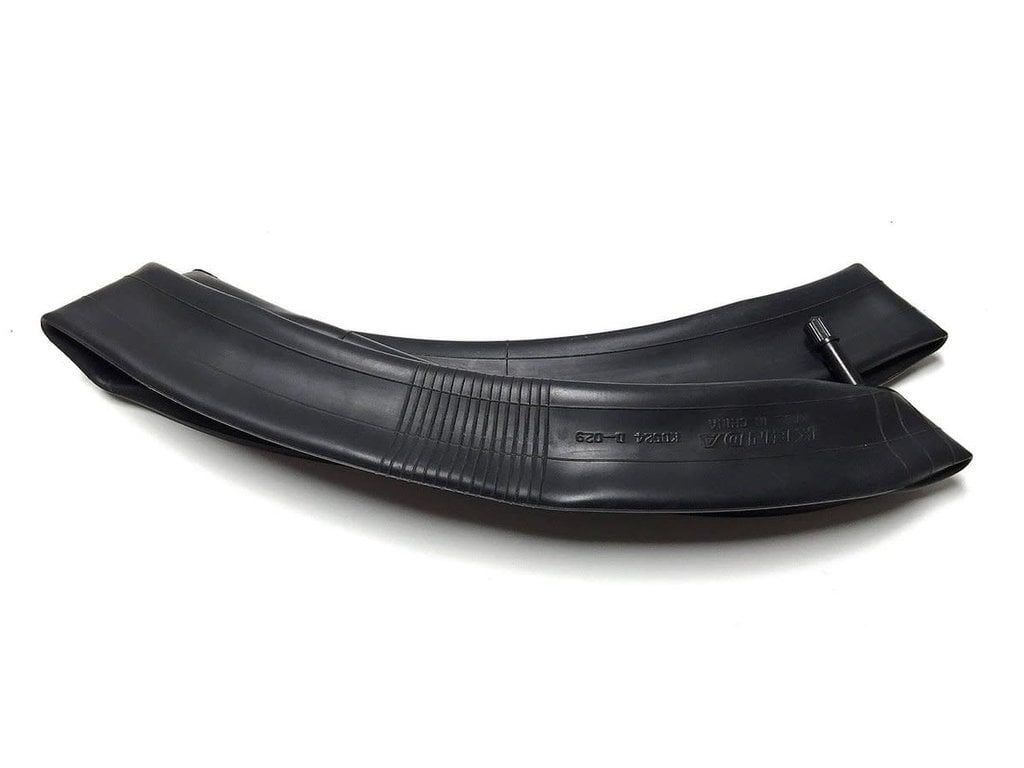The image depicts a deflated bicycle inner tube, folded into quarters against a solid white background. The black rubber tube is laid out in four overlapping sections, creating a layered appearance. The tube's air valve, which protrudes between the folded sections, is long and black with a distinctive white stripe down the middle and is silver-tipped. The tube also features some vertical ridges and embossed lettering, including a readable "D-029" and the partially visible brand name "KENDA, made in China." Subtle gray shadows cast by the tube add depth to the otherwise stark white backdrop.